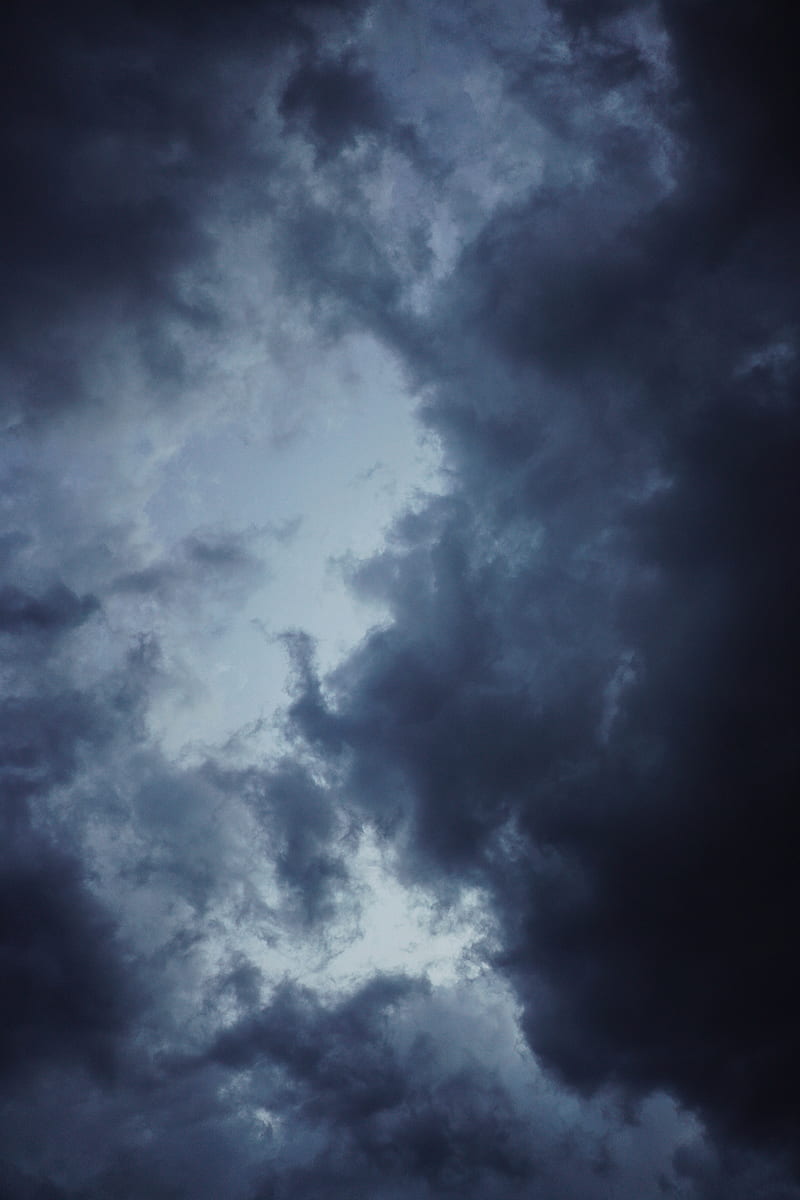This portrait-oriented photograph captures a dramatically cloudy sky, appearing dark and stormy. Thick, fluffy clouds dominate the frame, with a dark bluish-gray hue transitioning to nearly black at the edges, particularly in the top left and right corners. The sky is barely visible through small patches where the clouds part. In the center-left of the image, a gap in the dense clouds reveals a softer, light gray sky, giving the illusion of a faint glow, possibly sunlight. The photograph, taken from a bottom-up perspective, suggests either an overcast day or early evening, accentuated by the storm-like appearance and the overall gray-blue color palette. The clouds' wispy edges and fibrous texture add to the dramatic effect, making the scene look potentially digitally altered or AI-generated, though it retains the essence of a natural, heavily clouded sky.